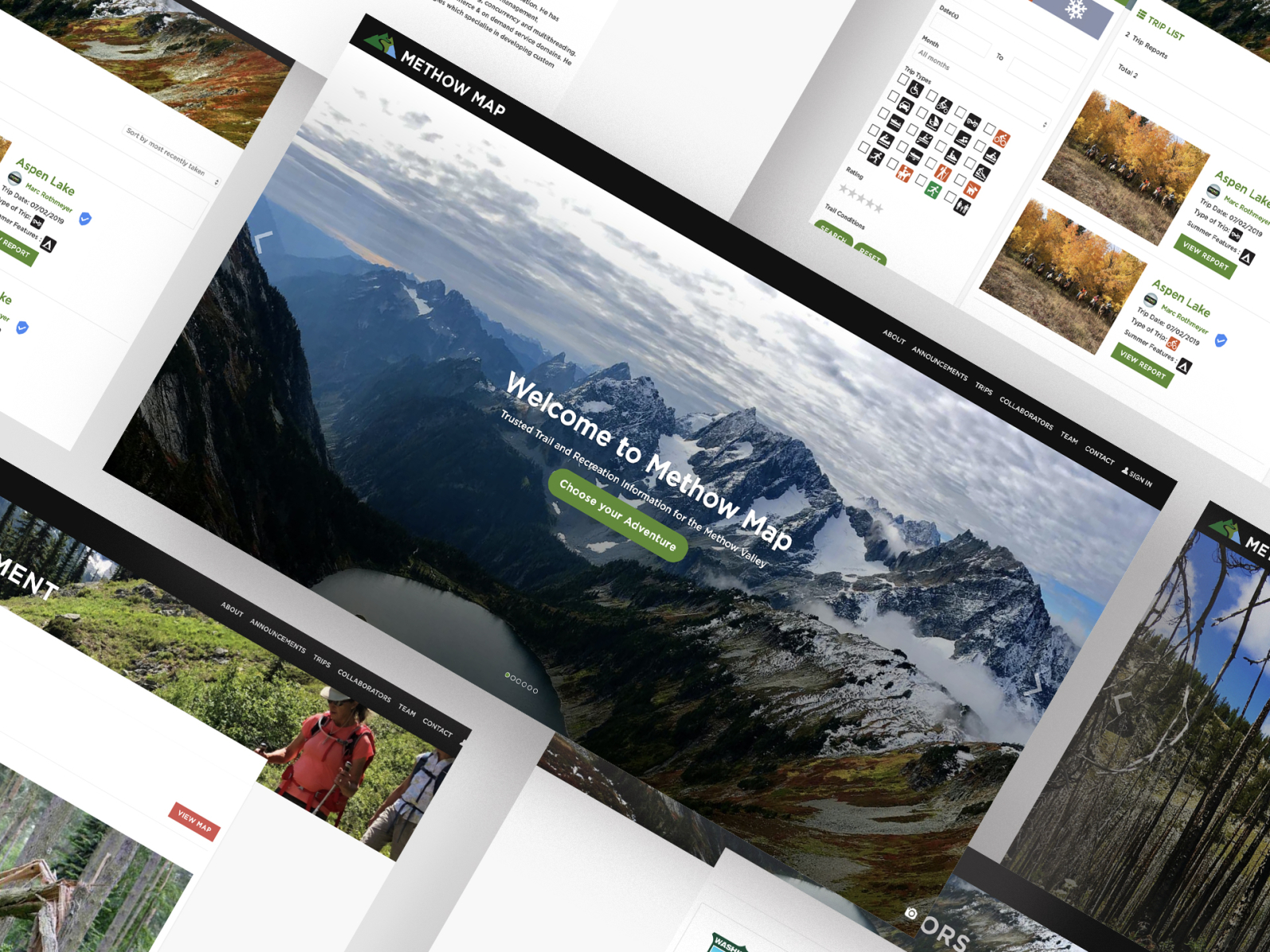The promotional image for the Methow Map website is artistically tilted on a diagonal axis, creating a dynamic visual appeal. Central to the image is a green and blue mountain logo with the text "Methow Map" prominently displayed beside it in clear, bold letters. A black border frames the top part of the main image. 

Positioned at the upper right corner, the navigation menu includes options such as About, Announcements, Trips, Collaborators, Team, Contact, and Sign In, making it easy for users to find essential information. The tagline "Welcome to Methow Map, Trusted Trail and Recreation Information for the Methow Valley" warmly invites visitors to explore the site.

In the center, the phrase "Choose your adventure" is highlighted, encouraging users to engage with the content. The background showcases an aesthetically pleasing scene of snowy mountains under a bright, cloudy sky, enhancing the overall attractiveness of the image. Surrounding the main visual are various snippets of pages related to hiking and camping, providing a glimpse into the adventurous opportunities available through Methow Map.